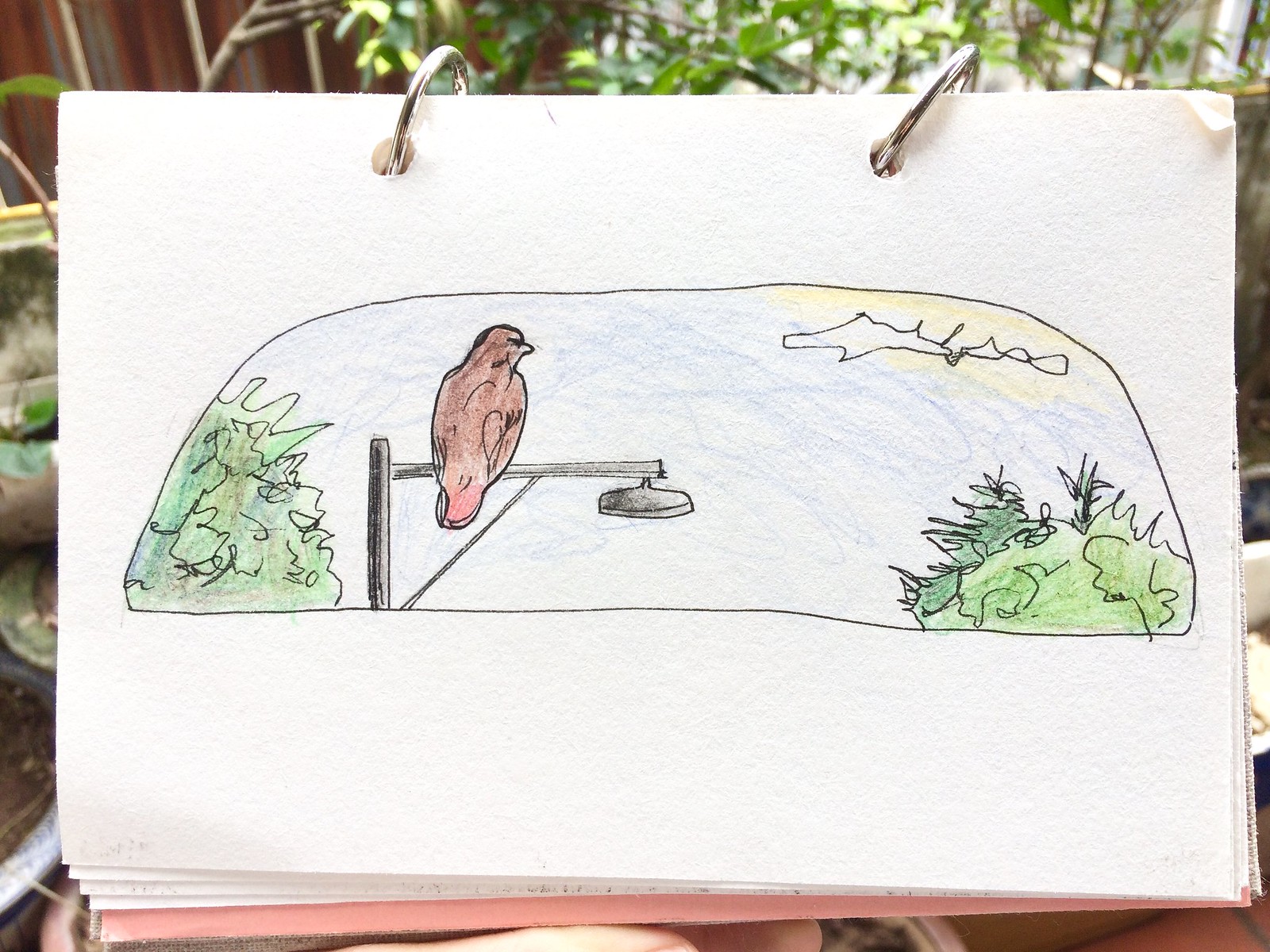In this outdoor scene, an artist is immersed in drawing, capturing the essence of nature in their sketchbook. The image, rendered on white paper within a spiral-bound sketchpad, is held open by silver rings with two visible holes at the top. Above the drawn scene in the upper right-hand corner, hints of sunlight pierce through the sketch, casting a gentle glow, though the sun itself remains unseen. Instead, the light cascades over green leaves and brown tree branches, suggesting an outdoor setting.

To the left of the image, a brownish wooden fence peeks through, and traces of soil are visible on both the left and right sides, grounding the scene further in an earthy environment. The central focus of the drawing appears to be an oval-shaped section, portraying a tranquil blue sky accentuated with whimsical, white, squiggly clouds. Verdant green bushes and towering trees frame the sketch, enveloping the scene in lush foliage.

At the heart of the drawing stands a black light post, capped by a light brown bird, adding a touch of life and vibrancy. The intricate use of colored pencils brings texture and depth to the composition, contrasting the vibrancy of nature against the simplicity of the sketchpad canvas.